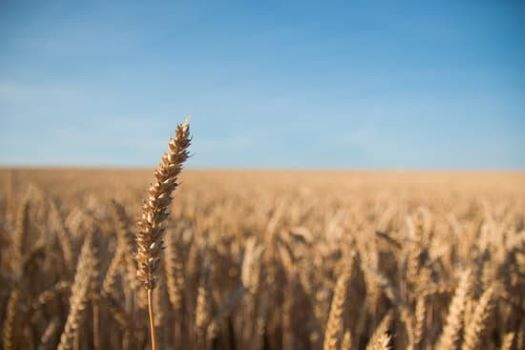The image captures a serene rural landscape during the late afternoon or early evening. In the foreground, a single stalk of wheat stands out prominently on the left side, its detailed beige-brown stalk adorned with seed casings contrasting sharply against a blurred sea of densely packed, golden wheat stretching horizontally across the field. Above, a vibrant Midwestern sky, characteristically deep blue with slight haze and patchy clouds, provides a bright, clear backdrop, enhancing the image's tranquil and expansive feel. The wheat field appears vast and overgrown, suggesting a setting where one could easily get lost amidst the towering stalks.